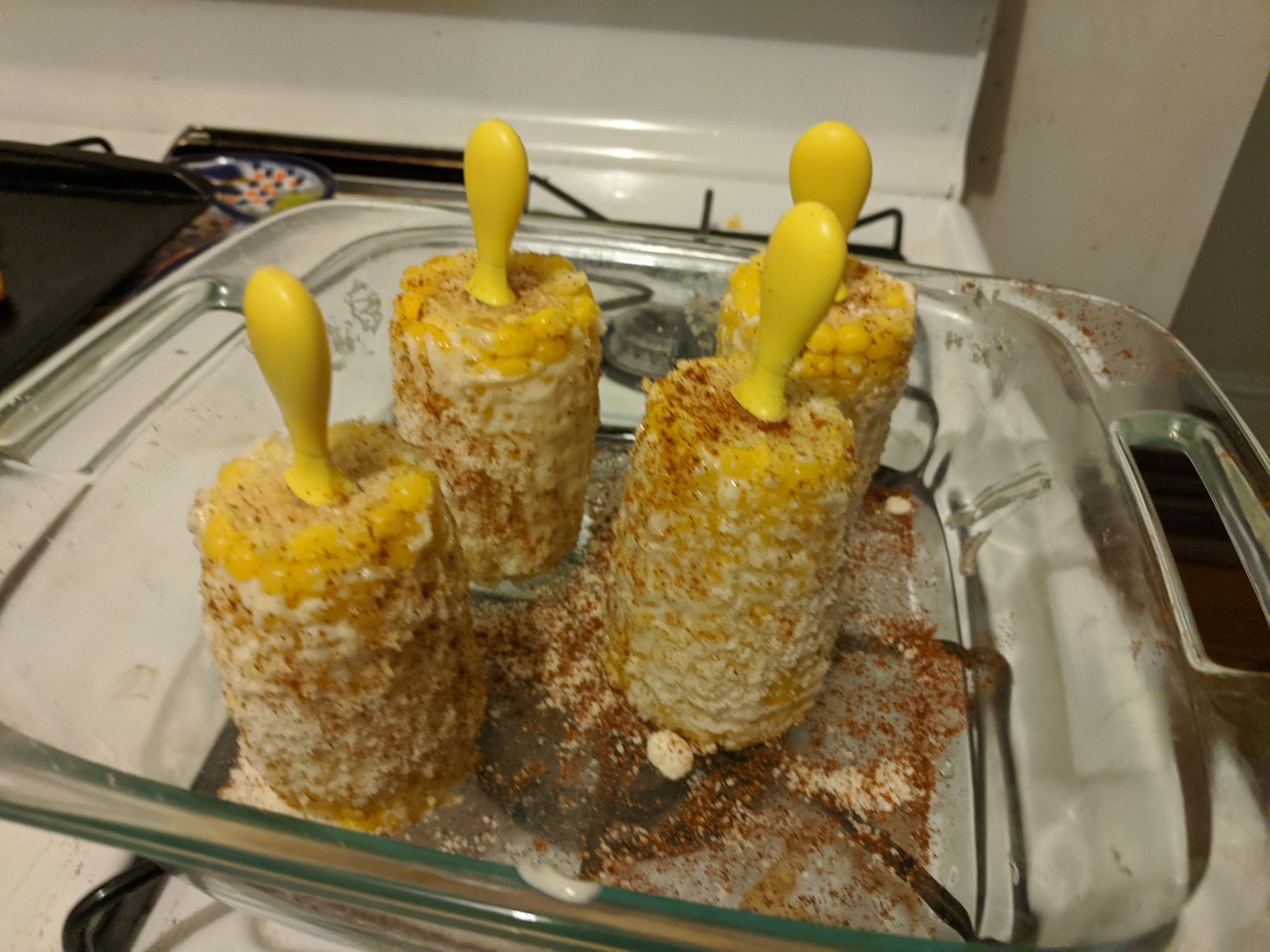The photograph captures a detailed close-up of a kitchen scene focused on the stovetop area. At the center of the image is a glass casserole tray with integrated handles, placed on a white ceramic hob. The circular hob has a metal frame, adding a subtle contrast to the white surface. Inside the glass tray, meticulously arranged, are four corn-on-the-cob pieces, each fitted with small, rounded yellow plastic handles resembling pacifiers. The corn is evenly coated with a butter-like substance and sprinkled with a red cinnamon-like seasoning, creating a visually striking layer of red dust atop the white gooey texture. The corns are arranged in pairs, with two at the front and two at the back of the tray. The composition is further framed by a black oven tray visible to the left and a blue-rimmed plate with a blue, red, and white pattern peeking out from the right side of the frame, enhancing the intricate yet homely kitchen setting.